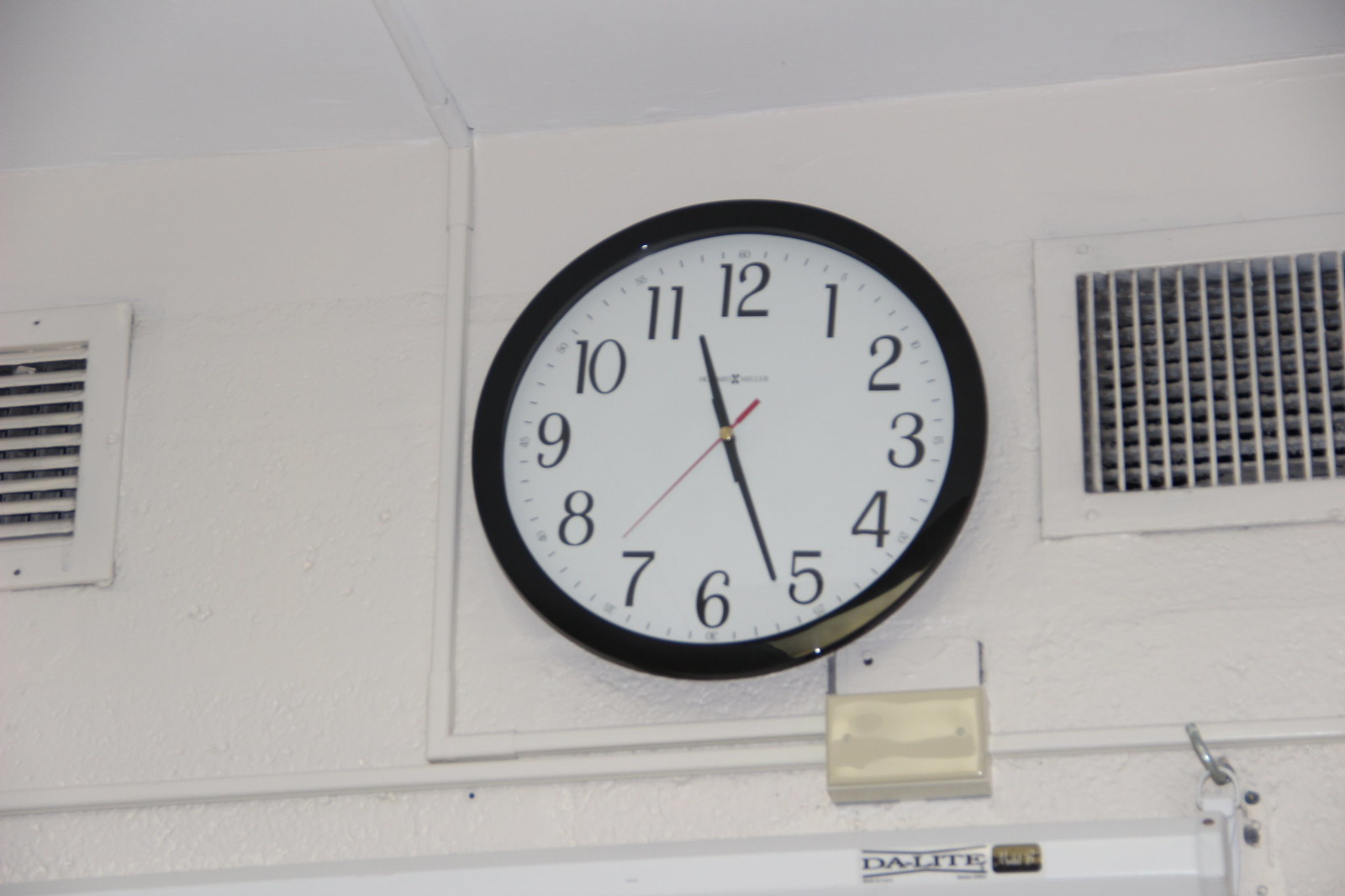This photograph captures an old-fashioned analog clock mounted on a white-painted cinder block wall, characteristic of older school buildings. The clock is black and white, with a distinctive red second hand pointing to the 37th second. The time displayed is 11:27. Positioned just below a retracted projector screen, which further suggests an educational setting, the image also features solid white ceilings. Additionally, a pair of air vents can be seen, aligning vertically with the clock, reinforcing the impression of a vintage school environment.